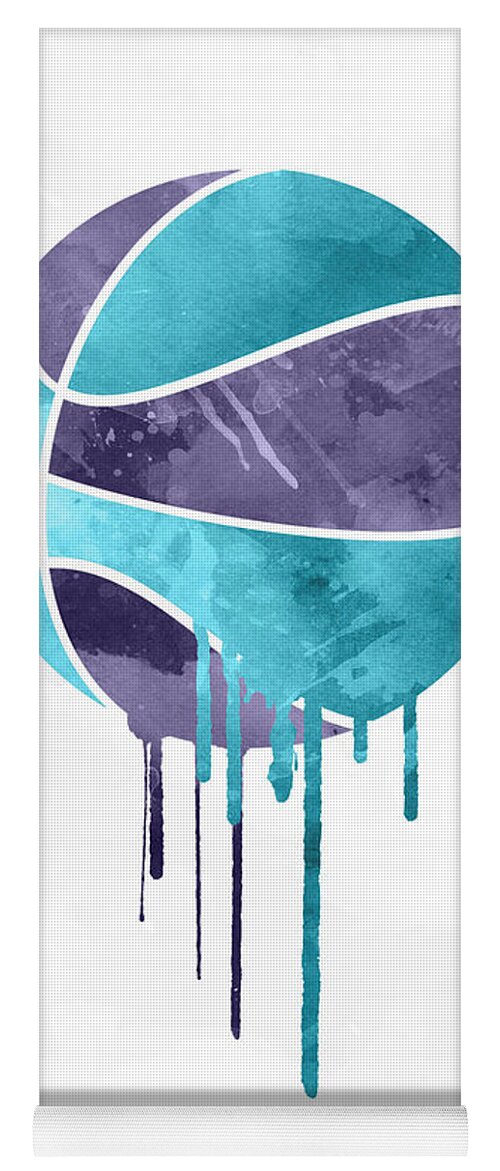The image depicts a painting on a tall, slim, white canvas, which gives the impression of a partially unrolled scroll or roller blind. In the center of the canvas is a round object resembling a basketball, yet uniquely painted in vibrant shades of purple and teal, instead of the typical orange. The ball is segmented by white lines and appears to be dripping paint downward, creating an artistic, fluid effect. The canvas or possible roller blind has a textured, canvas-like appearance, and the paint drips add dynamic motion to the otherwise static image. The background behind the ball is primarily white, adding contrast and emphasizing the colorful, dripping basketball. The entire canvas, which hangs vertically, does not fully display the basketball, as parts of it extend beyond the canvas edges. The bottom of the piece seems rolled up slightly, enhancing the impression of an unfinished, flowing work of art.